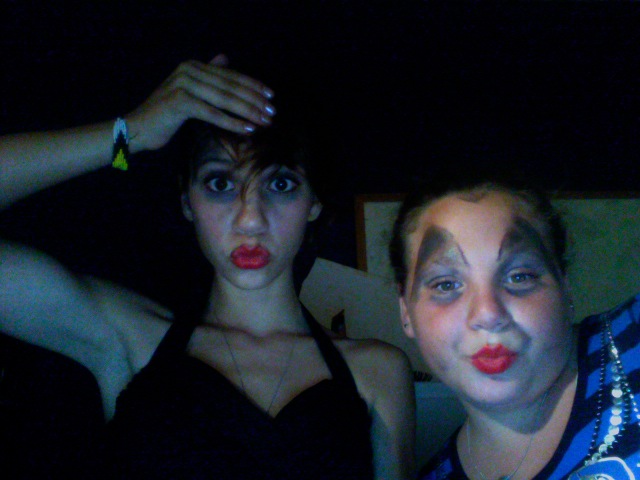In a dimly lit room with a black backdrop adorned with a few framed pictures, two individuals stand closely together, striking a pose. The first person, an older woman likely in her late 30s or 40s, is seen from the waist up, wearing a black halter top or strapless dress. She has short black hair and her makeup includes red lipstick, dark eyeliner, and mascara. Her lips are pursed in a duck-lip pose, and she extends her right arm, showing off a bracelet in black, yellow, and white beads, her silverish-painted fingernails gently running through her hairline.

Beside her is a younger girl, seemingly in her early teens, sporting a dark and light blue vertically striped t-shirt. She accessorizes with a black and silver beaded necklace. Her curly black hair is styled up, and she also wears red lipstick. Her face is painted with exaggerated, large black triangular eyebrows, and dark eye makeup, akin to clown makeup. Both individuals' eyes are wide open and emphasized by their heavy makeup, adding a dramatic flair to their expressions. The background is almost entirely black, except for a frame on the lower right side, which seems to contain a round object, possibly a map.